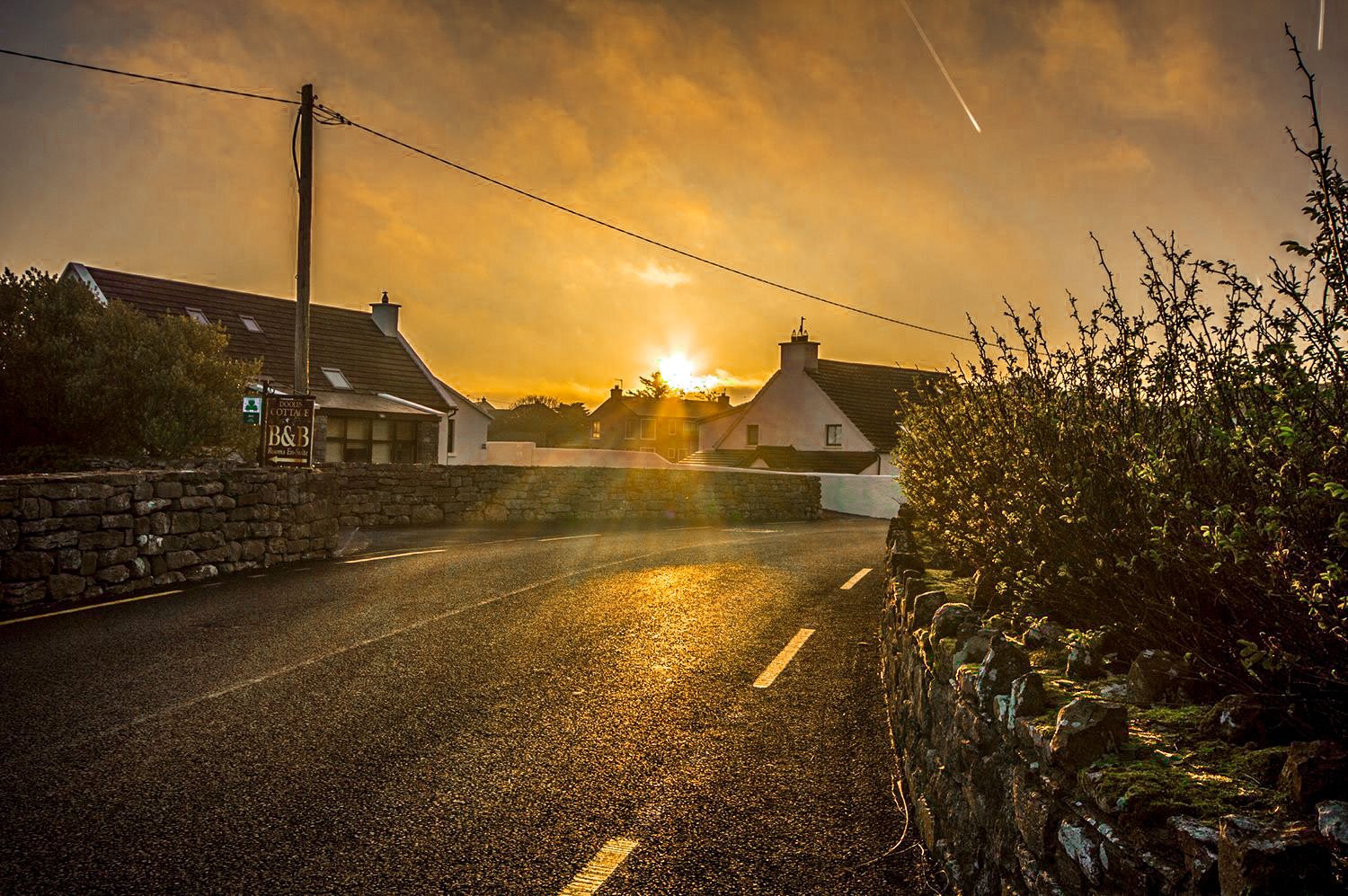The photograph captures a picturesque sunset over a quaint neighborhood, reminiscent of the English countryside. A well-maintained road with a yellow striped line runs through the scene, bordered by low stonework walls adorned with shrubs and greenery. Majestic crepuscular rays burst through the horizon, spreading a warm orange glow across the sky, which is streaked with clouds and contrails from passing planes. The road is flanked by two charming white houses with brown rooftops. One of these houses features a sign that reads "B&B." The sun is setting behind these structures, casting long shadows and illuminating the triangular rooftops. Telephone poles with power lines stretch over the homes, adding to the rustic charm of the setting. On the right side, the stone walls seem to sprout with plants, possibly corn or wheat, adding a touch of nature to the serene, orange-lit ambiance.